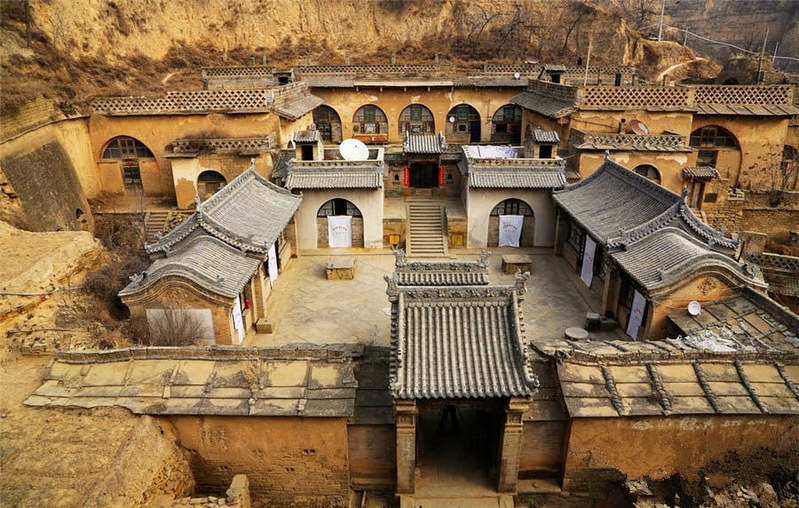This image depicts an overhead view of an ancient, possibly Chinese, village nestled in a rocky, mountainous area under an overcast sky. The terrain is covered with yellowish-tan rock and sparse brush, giving the scene a rugged ambiance. The village consists of modest homes and buildings, characterized by their creative, curvilinear roofs and ornate architectural features reminiscent of the Forbidden City in Beijing. White banners or towels hang from the windows and openings, adding a touch of mystique. 

Three significant, similarly colored buildings are positioned towards the back, accessed by steps. The foreground reveals smaller buildings, some with white banners draped from their entrances. There are distinctive, rounded, silver-gray roofs and arched windows, adding to the village's artistic charm. The area appears unkempt and possibly abandoned, with mud scattered throughout, suggesting it might have been affected by a mudflow. Despite its current state, the village's intricate design hints at its historical significance and past occupancy. An entryway provides access to the village, blending into the surrounding rocky structure, making the scene both picturesque and enigmatic.